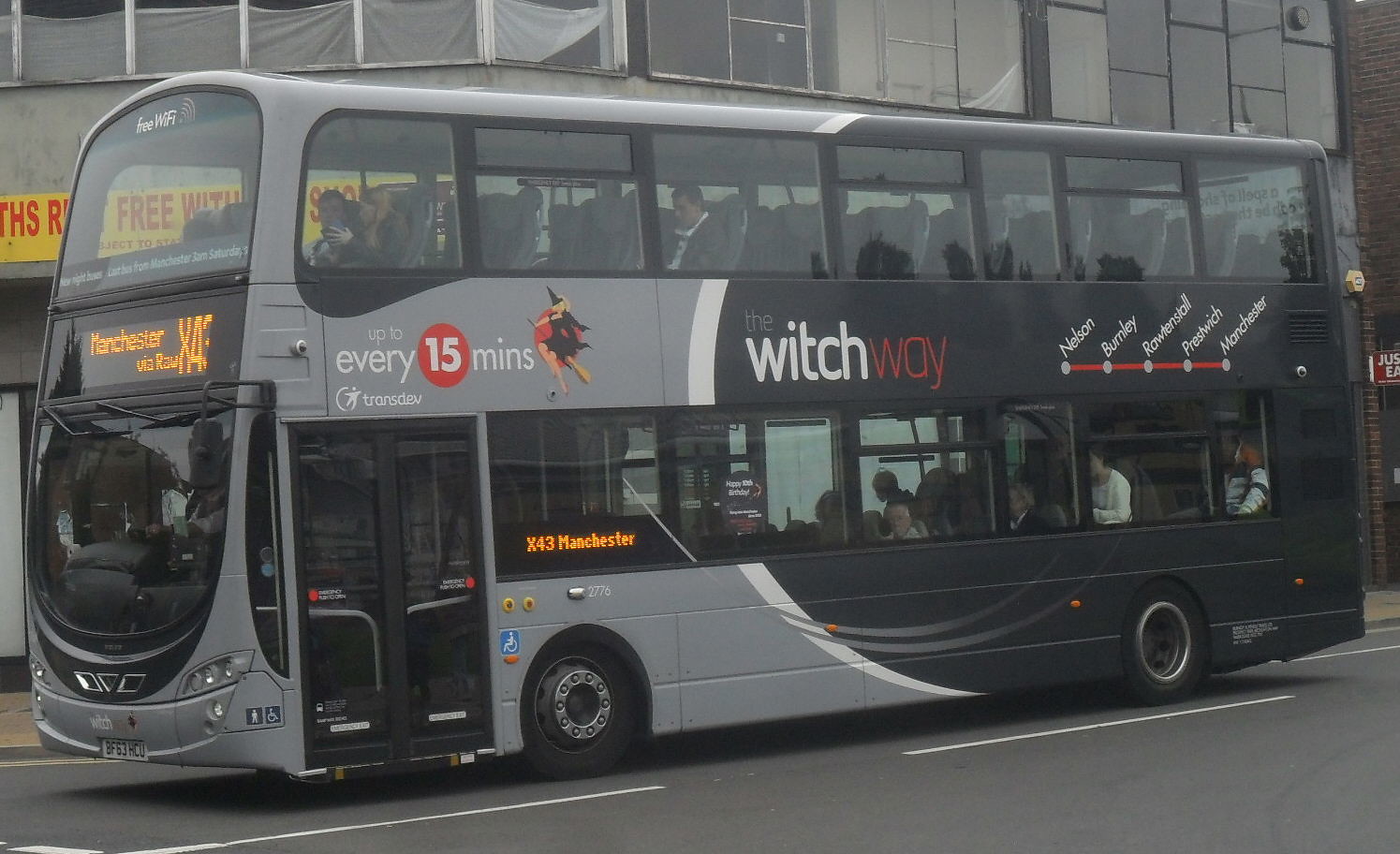The image showcases a double-decker bus traveling from right to left on a grey road. The bus is predominantly light gray on the front half and black on the rear half, with a thin white stripe running along its side. The front of the bus features a large glass window displaying the route "X43 Manchester." Above the driver’s window, there is a small screen indicating the bus's destination, Manchester, though some adjacent text is too small to discern. The side of the bus prominently displays the company's name, Witchway, alongside a small witch image and the text "every 15 minutes" in white. The entryway, located on the right front side, comprises black glass doors with small, unreadable text near the handles. Passengers are visible through the glass windows on both levels of the bus. In the background, a large building with numerous glass windows and a yellow sign with red writing adds to the urban scenery.